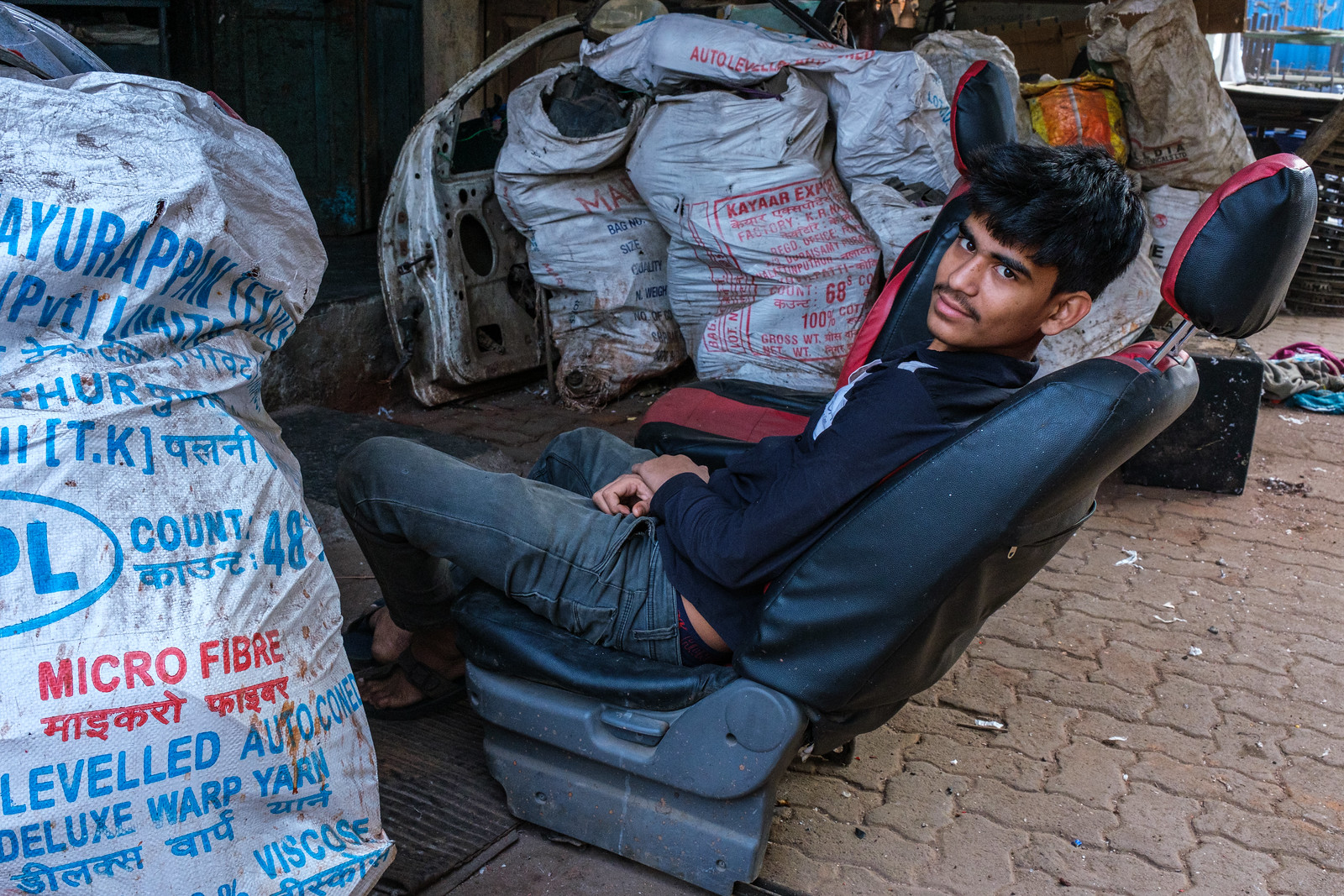In this photograph, a young man is sitting on a car seat that has been repurposed as a chair, positioned on a light-colored, reddish-brown brick sidewalk, possibly outdoors. The seat, which appears to be reclinable, features a distinctive design with black leather or vinyl on the exterior, red upholstery on the interior, and a gray plastic base. The seat lever is visible on the side, and a matching seat with red center stitching and black bolsters is present in the foreground. The man, who has short black hair and a mustache, is dressed in a black long-sleeved shirt with white detailing on the chest and jeans. He is leaning back, smirking slightly as he looks towards the camera.

Surrounding him are several large, dirty white plastic sacks filled with unspecified contents, marked with both blue and red lettering, partially in English and a foreign script that appears to be Hindi. The area around him is cluttered with debris and trash, contributing to the overall unclean appearance of the setting. In the background, a grimy white car door rests against a wall, further adding to the disarray.